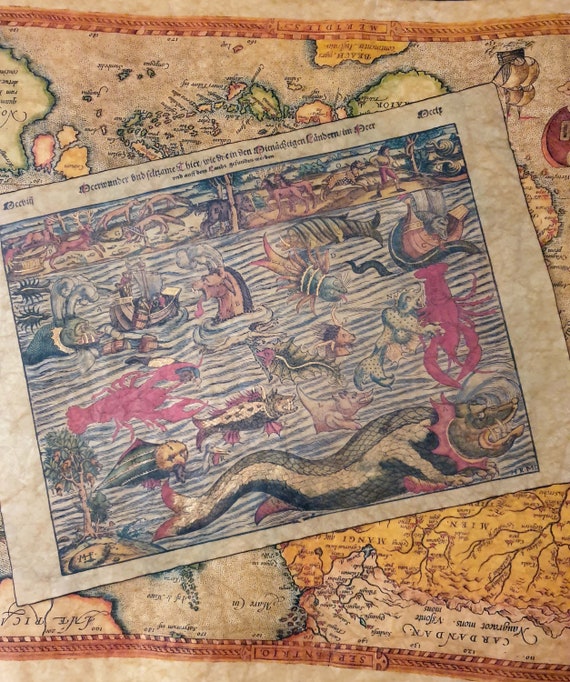The image features an ancient world map displayed on a large, floor-covering rug with a brown border. The map itself is upside down, with North America positioned in the bottom right corner and its countries rendered in light, watercolor-like hues. Overlaying the map, there is a vivid illustration bordered with black and white lines, making it look like an old piece of parchment. This additional layer depicts fantastical sea creatures and monstrous beings. Among the prominent figures are a colossal lobster with a human figure in one of its claws and various other sea monsters, including one at the bottom of the image and another at the top, the latter with its tongue sticking out. Additional details include creatures bothering a boat resembling a Chinese junk, lands at the top featuring coyotes, horses, and a man with a stick in the upper right corner. The word "cardanden" appears in the lower right, hinting at the map's ancient origins. The overall scene is intricately detailed, capturing a sense of historical adventure and mythical intrigue.